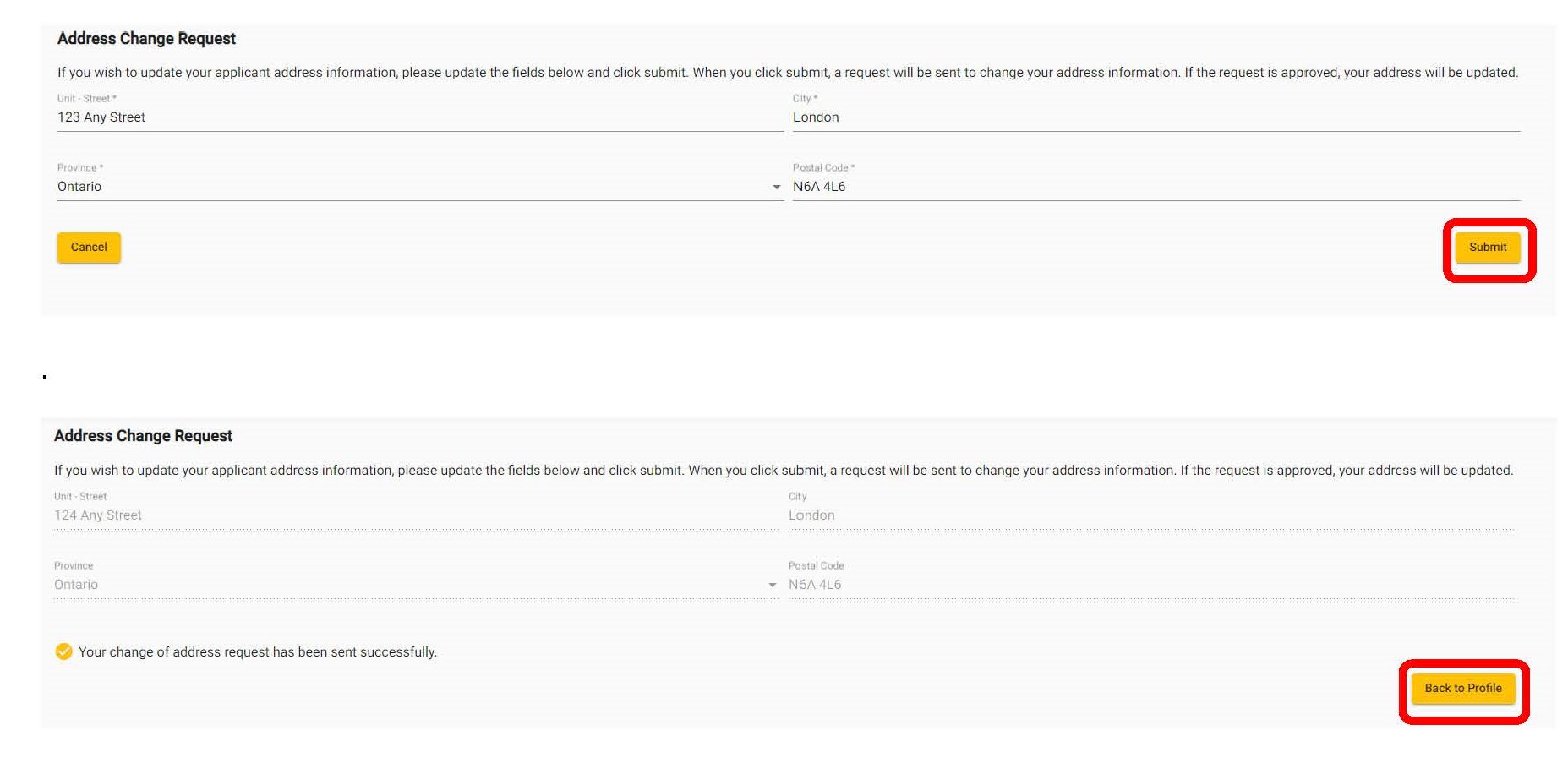The screenshot showcases two rectangular images of address change request forms, cropped and edited into a single visual. The first form, positioned at the top, displays the heading "Address Change Request" in bold font on the top left. Beneath the heading, instructional text reads: "If you wish to update your applicant address information, please update the fields below and click submit. When you click submit, a request will be sent to change your address information. If the request is approved, your address will be updated." 

This form includes four text fields designated for the street, province, city, and postal code. At the bottom of this form, there are two buttons: a "Cancel" button located on the bottom left and a "Submit" button on the bottom right, highlighted by a red box edited around it.

The second form, placed below the first, mirrors the layout and text fields of the initial form. However, at the bottom left, it features a message that reads: "Your change of address request has been sent successfully," accompanied by a yellow circle with a white check mark in the center. To the right of this message, a "Back to Profile" button is displayed, also highlighted with a red box edited over it.

The two images function as a before-and-after set: the first image illustrates the address change request form prior to submission, and the second image shows the page's confirmation screen after the request has been submitted.